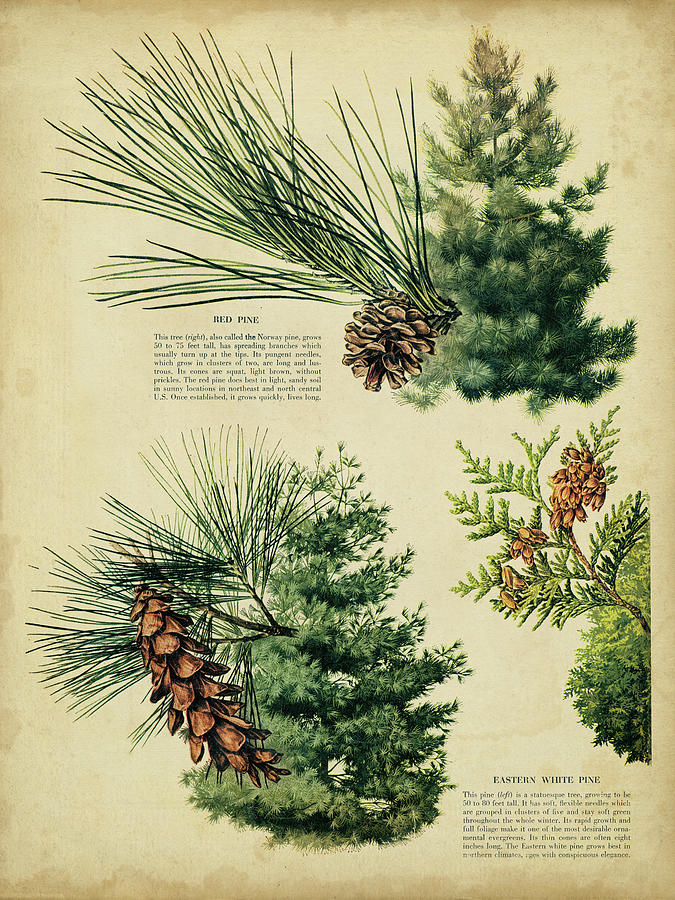The image is a detailed page from an old botanical book, showcasing various types of pine trees, likely including red pine and eastern white pine. The page appears weathered, enhancing its vintage aesthetic. Central to the page are three distinct, hand-drawn or digitally printed illustrations of pine trees with corresponding pinecones. The colors range from light green to dark green, brown, and light brown, set against a beige background. The top right corner features an illustration labeled "red pine" with green letters, while the bottom center highlights an "eastern white pine," also in green text. Each tree illustration is accompanied by a close-up of its respective pine leaves, displaying little spikes. Two paragraphs of explanatory text are positioned in the top left and lower right corners, though the font is too small to decipher. The entire composition is brightly lit, giving it a crisp and clear appearance, despite the tiny, unreadable lettering.